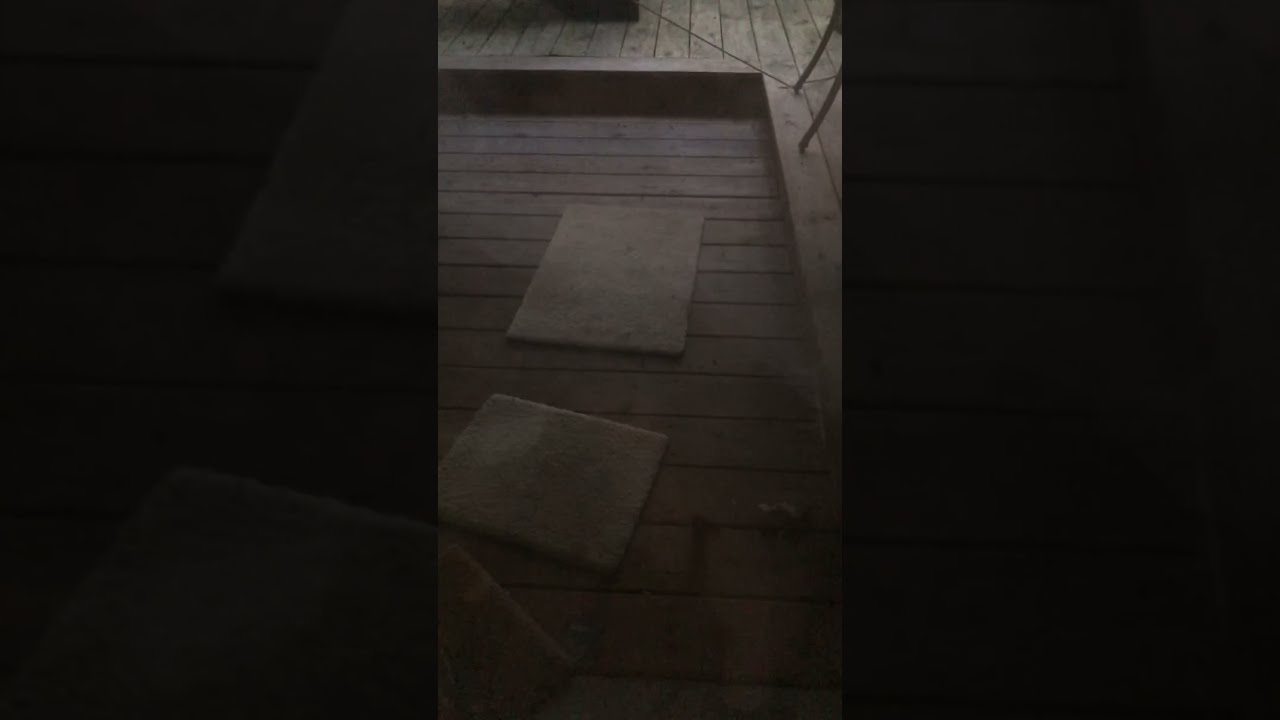The image depicts a dimly lit, possibly outdoor setting, with the left and right sides shrouded in darkness. At the center, there lies a wooden deck made of planked wood with a tannish or faded brownish hue. The mid-section of the deck features two carpet squares—one located in the bottom left and another directly above it, complemented by a longer carpet strip in the center. These carpets appear to be beige with some signs of wear or dirt. There’s an elevated portion, resembling a step, leading to a vertically patterned extension of the floor on the top left, marked by various circles and off-colored blemishes. In the background, cut off by the surrounding darkness, there appear to be short poles or chair legs in black, hinting at outdoor furniture. No text or writing is present, emphasizing the stark and somewhat mysterious nature of the dimly lit porch area.